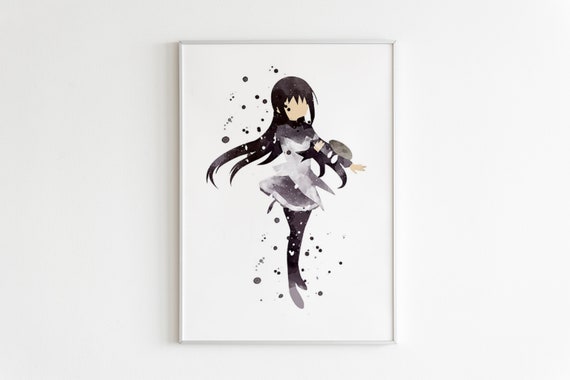This image features a detailed painting of a faceless young female figure in an anime style, framed inside a simple, straight white frame. The artwork is set against a pure white background, with a noticeable light source shining from the right. The female character is distinguished by her long, dark black hair and monochromatic clothing in shades of gray and black. She is adorned in a short dress paired with pants or leggings, and her outfit is patterned with scattered black polka dots. Notably, she seems to be interacting with a device on her left arm using her right hand. Surrounding her are various colored or black circles, which might represent some form of energy or superpower. This stylized figure, with thematic elements and no facial features, is positioned directly on the white wall without any accompanying text.